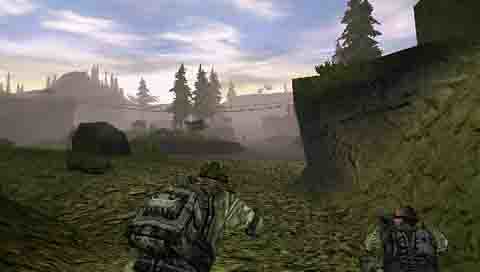The image is a wide screenshot from a retro video game, likely SOCOM, characterized by its third-person tactical shooter perspective. The scene is set outdoors during the day, under a partly cloudy blue sky that fades into a hazy, foggy background. Along the horizon and throughout the landscape, patchy clusters of pine trees can be seen, with some trees more prominently near the foreground, including a notable pine on the right. The terrain consists of a mix of grass and dirt, featuring a hillside on the right. In the foreground, two figures dressed in army camo with backpacks and helmets are visible: one positioned just left of center, visible from the waist up, and the other in the lower right corner, seen from the mid-torso up. The image has a blurry, low-resolution quality, typical of older video games, and lacks any textual elements. There also appears to be a faint outline of a building in the distant background, contributing to the overall hazy and distorted appearance of the scene.